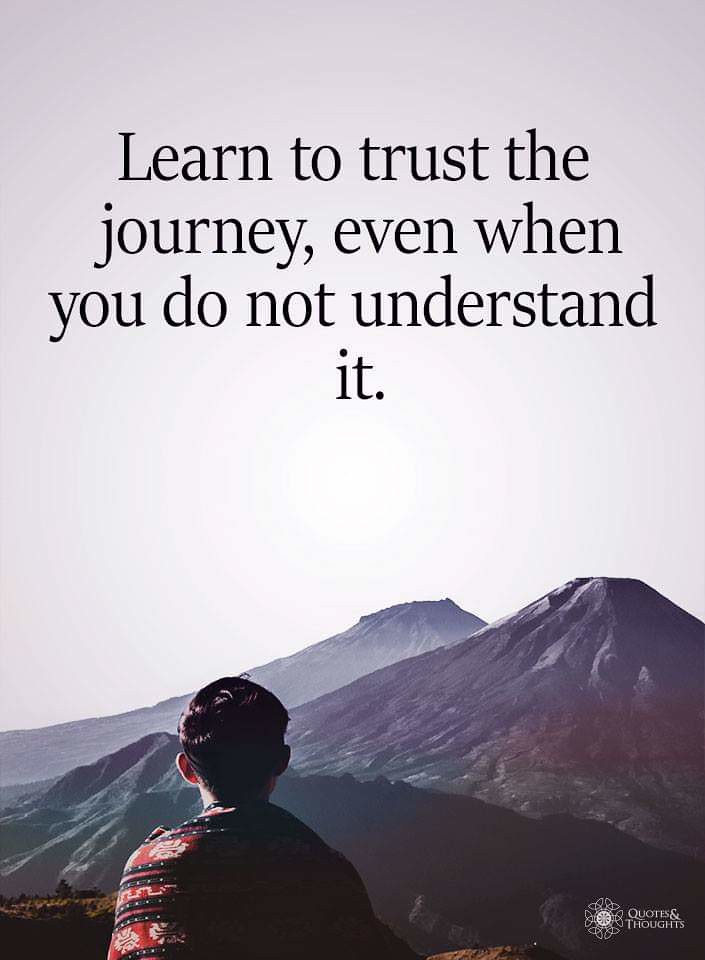The image features a singular object: a poster that fills the entire frame. The poster showcases an inspirational quote in the center, spread across four lines of black text: "Learn to trust the journey even when you do not understand it." The background is an outdoor scene captured in daylight, predominantly displaying an open sky. Centrally positioned in the image, a boy with short black hair, draped in a red and black blanket adorned with white flowers, gazes towards a mountain range on the right. In the bottom right corner of the poster, a geometric flower logo appears, accompanied by the text "quotes and thoughts" in white. The color palette includes tans, blacks, grays, reds, maroons, and whites. The overall composition emphasizes the journey theme, enveloped in an outdoor setting that fosters a sense of contemplation and inspiration.